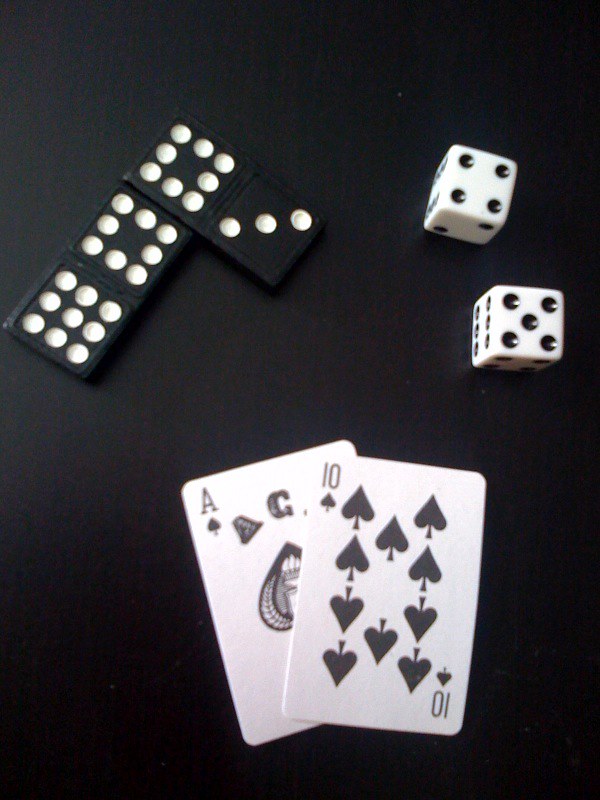In the image, set against a black background with a matte to semi-glossy finish, there is a table or desk that features several gaming pieces strategically placed. In the top left corner, two black and white dominoes are positioned; one domino shows eight circles on one side and three on the other, while the second one displays eight circles on one side and nine on the other. In the top right corner, two white dice with black dots are present; the upward-facing sides display four and five, while the visible sides of the bottom right die reveal four and six and the sides of the top die show the two. At the very bottom of the image, there are playing cards: a white ace of spades and a ten of spades, both face-up. The ten is slightly angled and overlapping the ace.